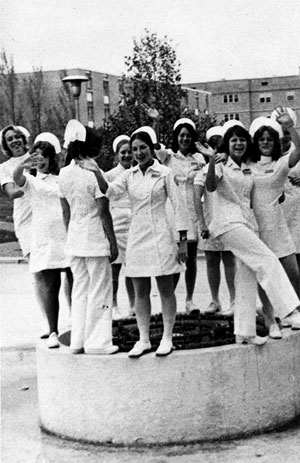This black and white vintage photograph captures a celebratory group of about 12 women, all dressed as nurses in traditional uniforms from the 1960s to 1970s, standing on a circular stone planter filled with mulch. The nurses are uniformly attired in white, with their distinctive caps; some wear knee-length dresses paired with white heels, while others don slacks and white shirts. They appear joyous, with several waving, hugging, and one even kicking her leg out playfully. Behind the group stands a tall tree that towers over the nurses, and in the background, a large brick building—likely a hospital or school—is flanked by a couple of smaller trees and a street lamp. The central figure, a nurse smiling and waving directly at the camera, underscores the exuberant mood captured in this timeless photograph.